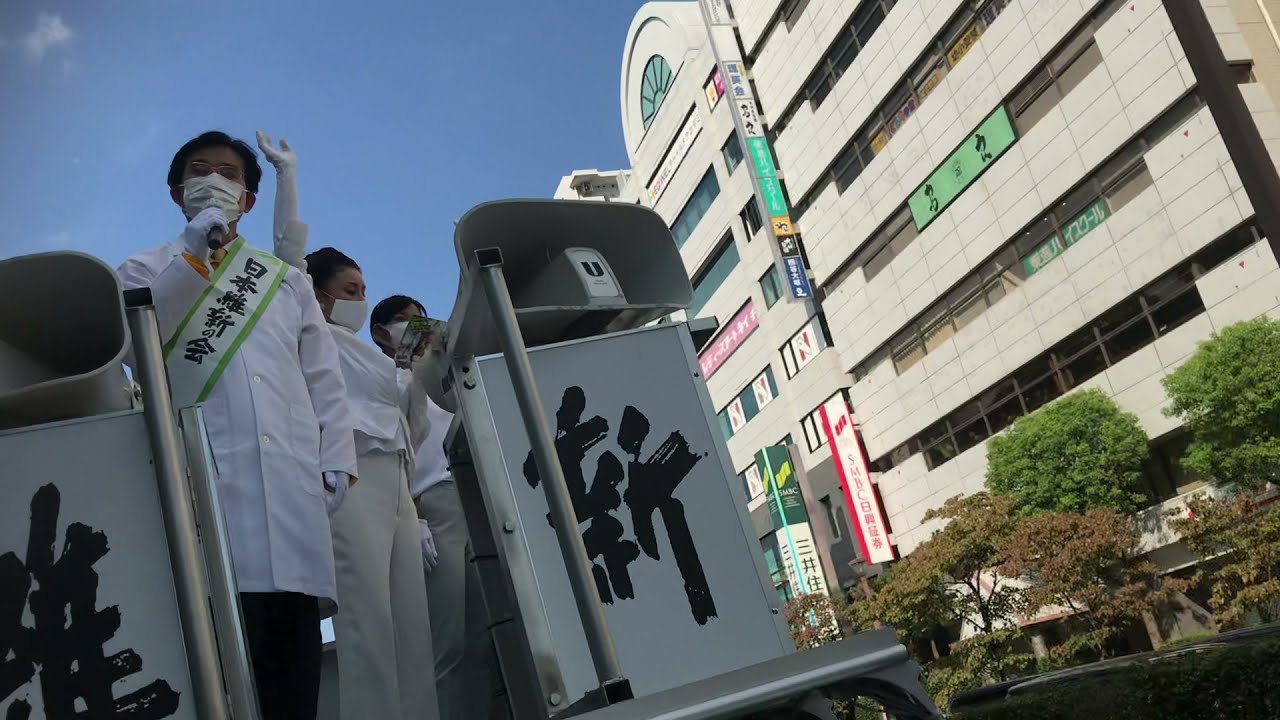In this vibrant outdoor scene, several masked individuals stand near a white, double-decker bus-like vehicle adorned with black Asian characters against a grey background. The man on the left is dressed in a white lab coat with black pants and wears a green and white sash featuring Asian writing. He holds a microphone. Beside him, a woman in a white shirt and khakis raises her right hand, while another woman stands next to her in similar attire. The background showcases a large, white, multi-story building, possibly a hospital, decorated with colorful billboards and signs in green, blue, yellow, pink, white, and red. The building has numerous windows, and the scene is lit by a mostly clear blue sky with a few clouds in the upper left corner. To the right, there are green and brown plants and trees, adding a touch of nature to this urban setting.